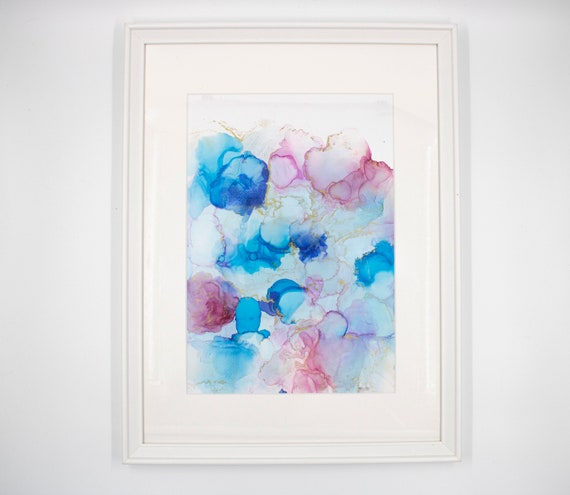The image is a close-up photograph of a square watercolor painting hanging on a white wall. The painting is set within a white canvas, enclosed by a white border, and framed with a white frame, giving the entire presentation a refined, modernistic elegance and simplicity. The artwork itself contrasts elegantly with its surroundings, featuring an abstract design that resembles a combination of flower petals or fluffy clouds. The colors in the painting are primarily hues of deep blue, light blue, and purple on the left side, transitioning to reddish and purplish tones on the top right, with subtle touches of yellow and fine gold lines intermingled. The overall composition exudes a subtle yet striking vibrancy against the clean white backdrop.